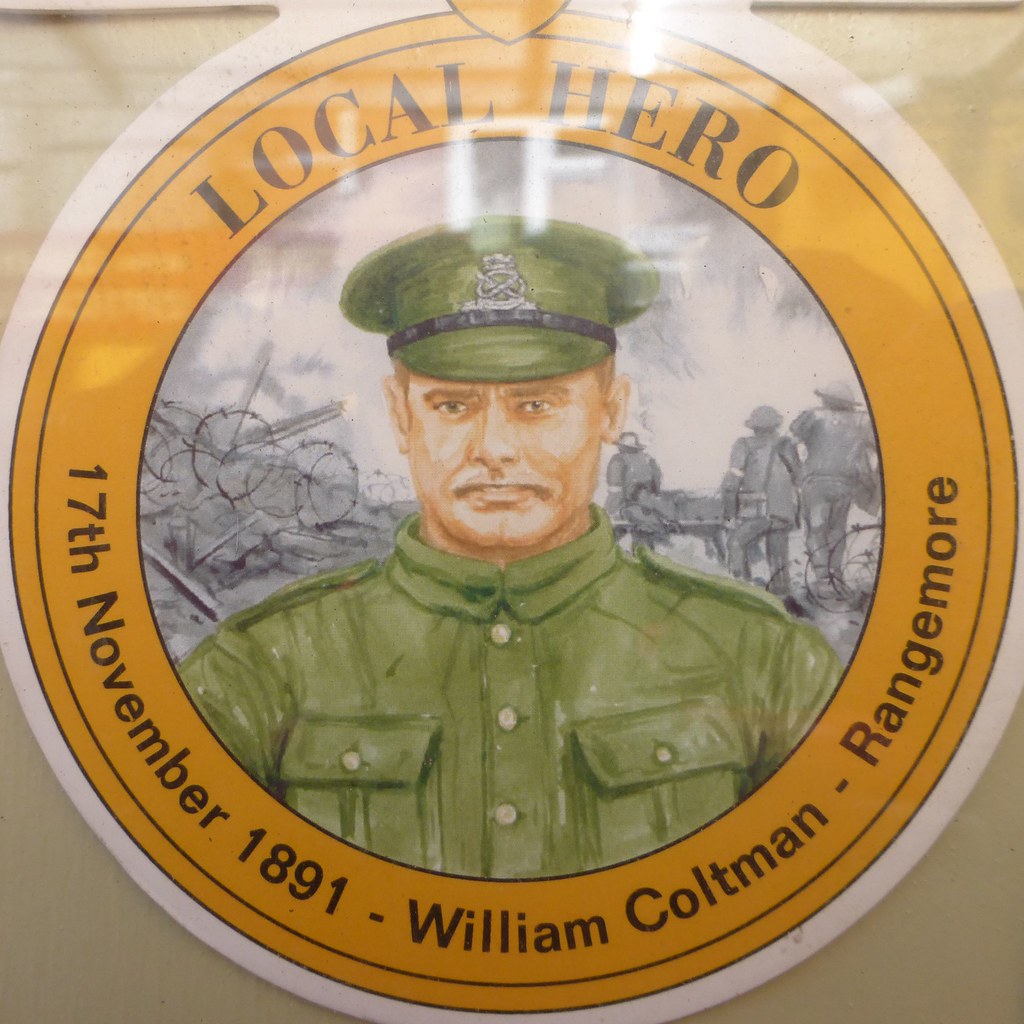The image depicts a prominently featured cartoon-style drawing of a white male soldier with a mustache, centered within a reflective yellowish-orange circle, bordered by a white rim and positioned against a tan background. The soldier, wearing a green military uniform with a three-button placket, collar, two flap chest pockets, and shoulder epaulets, gazes directly at the viewer. His green hat bears a silver emblem. Surrounding him, black-and-white wartime scenes illustrate men in hard hats carrying stretchers and a bunker protected by barbed wire. The top and bottom of the circle feature black text that reads, "Local Hero, 17th November 1891, William Coltman, Rangemoor," commemorating the soldier's historical significance.